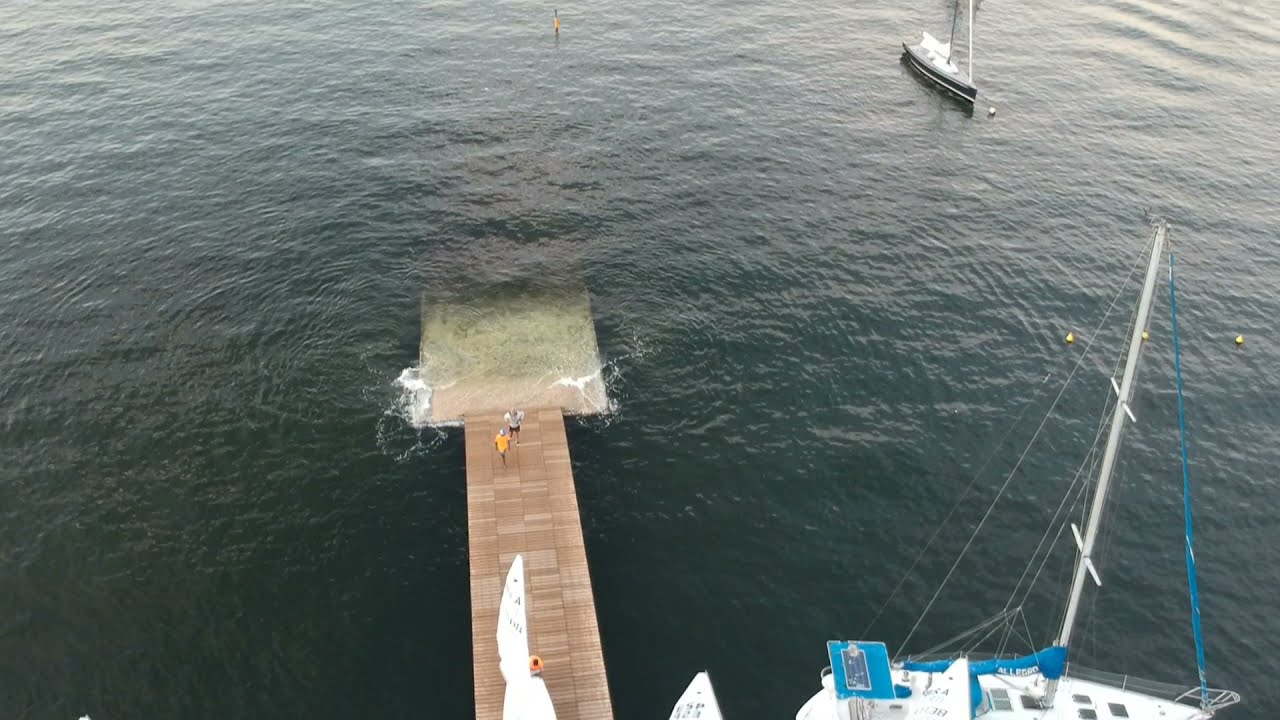The image is a color photograph taken from a drone, presenting a detailed top-down view of a sailboat launch area in an ocean setting. In the lower foreground, a white sailboat with a blue sail cover sits prominently, its sails down. Adjacent to this boat, on the lower left, is a wooden ramp projecting from the bottom of the image, extending outward and dissolving into the bluish-grey, somewhat dull water, which is marked by soft, small ripples. Two individuals, one in a yellow shirt and the other in a white t-shirt, are visible standing near the end of the ramp, appearing distant and indistinct. In the upper right of the image, a smaller black and white sailboat is seen, also with its sail down. The scene is captured in a photographic style of realism, emphasizing the mundane yet serene details of the boat launch area.